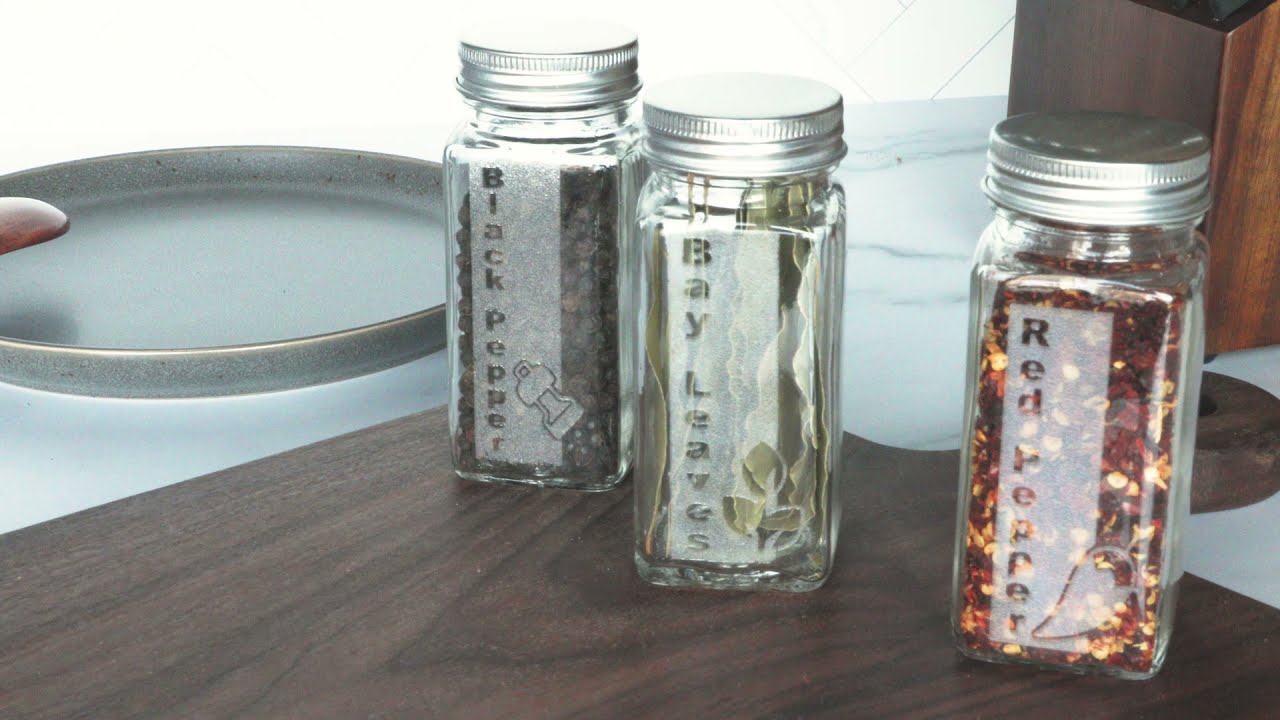This photograph beautifully captures an assortment of three spice jars arranged on a dark-stained wooden cutting board, set against a kitchen counter backdrop. The jars, positioned towards the right center of the image, are elegant rectangular glass containers, each topped with a sleek silver cap.

1. **Red Pepper Jar**: The jar on the far right showcases a vivid array of dark red and tan red pepper flakes, visible through its transparent sides. The label, "Red Pepper," is boldly displayed vertically along the side.
 
2. **Bay Leaves Jar**: At the center, the jar filled with aromatic bay leaves features a similarly vertical label, "Bay Leaves," embossed on its glass surface. Its leafy contents add a touch of green to the composition.

3. **Black Pepper Jar**: To the left, the third jar holds a generous portion of whole black peppercorns. Like its counterparts, the label, "Black Pepper," is elegantly etched vertically on the side.

To the left of the Black Pepper jar, a sleek black and shiny tray—or perhaps a plate—adds a contrasting element to the scene. In the background, a dark-stained wooden box provides a rustic touch, enhancing the overall warm and earthy palette of the image.